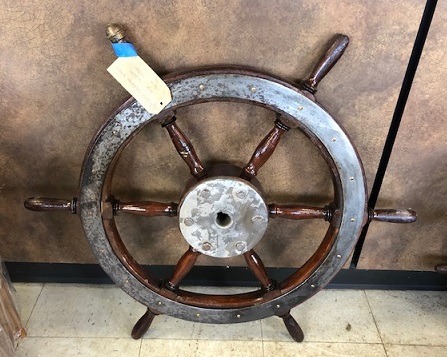In the photograph, a dark brown, wooden ship's steering wheel with six handles is prominently placed against a wall. The wheel, which features a white label with blue tape attached, exhibits signs of age with a shiny but worn surface. It rests on a cream-colored tile floor that appears dirty and slightly grimy. The backdrop is a wall displaying various shades of brown. The circular center of the wheel is hollow, giving it an aged and somewhat neglected appearance.